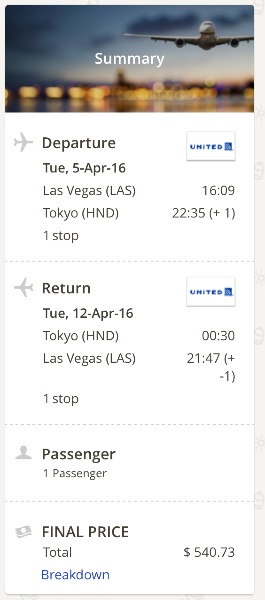The image depicts a vertically oriented screenshot, likely from a mobile app or website, with dimensions approximately three times its height compared to its width. 

At the top of the image is a main banner featuring a scenic backdrop of either a sunrise or sunset over the sea, with an airplane landing towards the viewer's direction on the right-hand side. Overlaying this banner, centered in white text, is the word "Summary."

Below the banner, the screenshot is divided into two main sections: one for departure and one for return, each taking up about half of the remaining space.

**Departure Section:**
- At the top, a gray airplane icon faces right.
- "Departure" is noted.
- The date "Tuesday, 5th of April, 2016" appears.
- Following this, the departure and destination locations are listed:
  - "Las Vegas (LAS)"
  - "Tokyo (HND)"
- It is indicated that there is "one stop" during the journey.
- On the right-hand side:
  - A United Airlines logo is displayed.
  - The departure time from Las Vegas is "16:09."
  - The arrival time in Tokyo is "22:35 (+1)."

**Return Section:**
- Mirroring the layout of the departure section, a gray airplane icon here faces left.
- "Return" is specified.
- The date "Tuesday, 12-APR-16" is given.
- Below the date, the same airport codes are used to indicate the return flight from Tokyo to Las Vegas.

Overall, the screenshot provides a concise summary of an upcoming round-trip flight between Las Vegas and Tokyo, noting key details such as dates, times, and the airline involved.